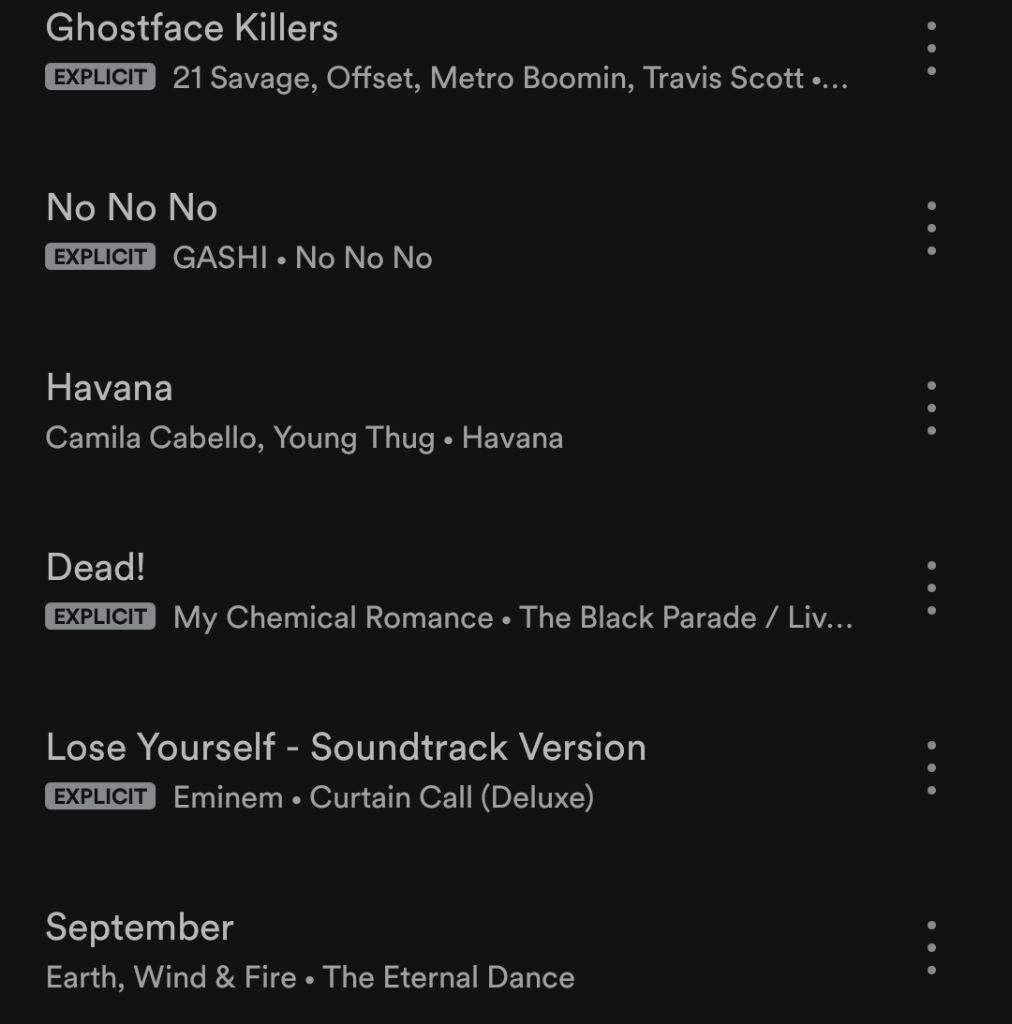This is a screenshot of a portion of a Spotify playlist featuring a black background. Each song listed has a vertical ellipsis (three dots) on the right side for additional options. The text is white, and several of the tracks are labeled with an explicit content warning.

1. "Ghostface Killers" by 21 Savage, Offset, Metro Boomin, and Travis Scott has an explicit content warning.
2. "No No No" by GASHI also features an explicit content warning.
3. "Havana" by Camila Cabello featuring Young Thug is marked with an explicit content warning. 
4. "The Black Parade / LIV" by My Chemical Romance includes an ellipsis indicating additional text or details.
5. "Lose Yourself (Soundtrack Version)" by Eminem from the album *Curtain Call (Deluxe Edition)* is tagged with an explicit content warning.
6. "September" by Earth, Wind & Fire from the album *The Eternal Dance* is listed without an explicit warning.